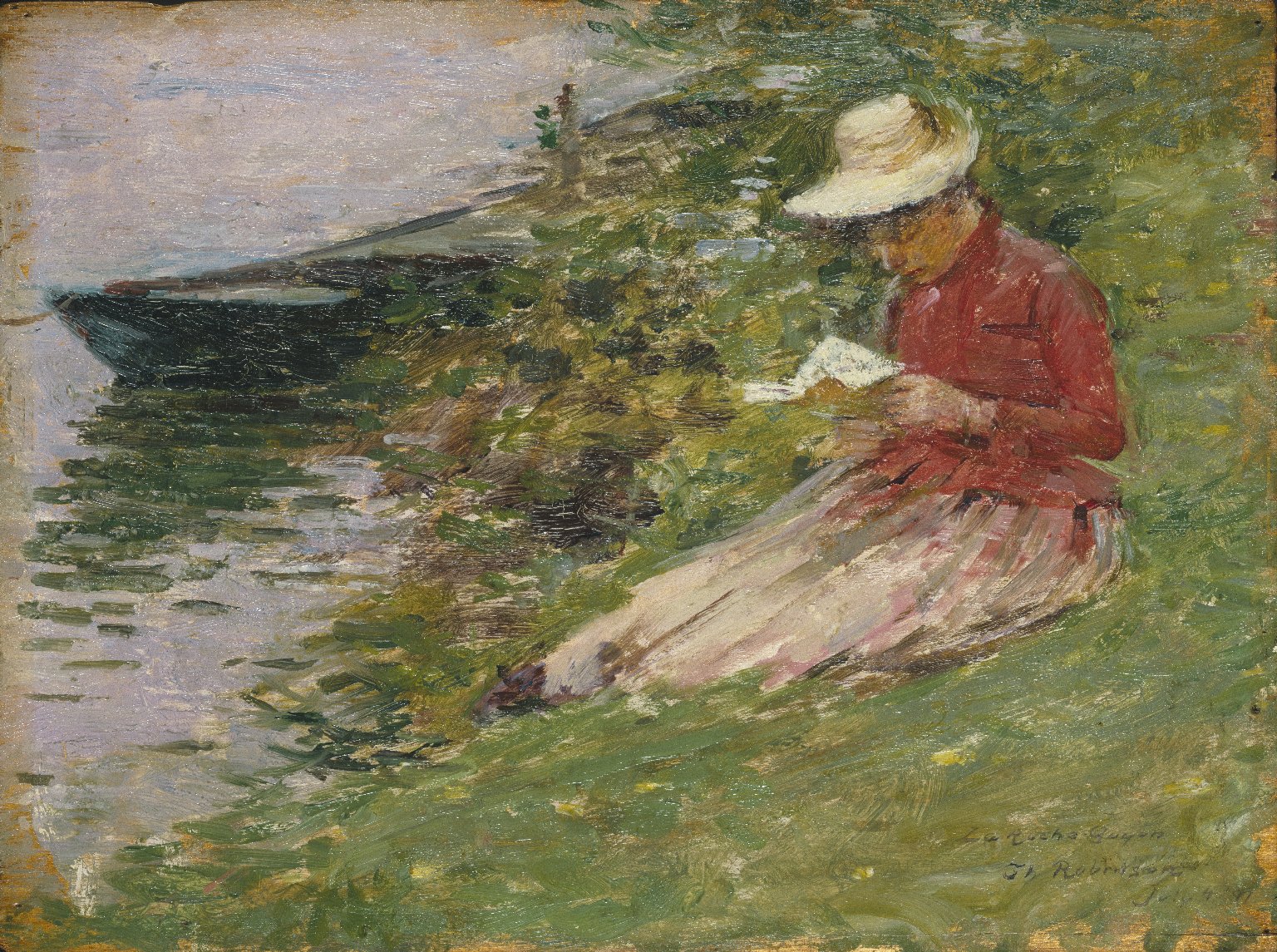The impressionist oil painting depicts a serene scene by a body of water, extending from the upper left to the lower left corner of the image. A lone canoe, casting a shadow and a reflection on the water's surface, is tied off with a rope. Seated close to the edge of the water on an olive green and yellow-splotched grassy hillside is a woman absorbed in a book. She wears a yellow sun hat, a high-necked red long-sleeve top, a white full skirt, and black shoes. Her legs are extended in front of her as she sits in a patch of smoother grass. The texture of the brushstrokes is visible, adding depth to the scene. In the lower right-hand corner, there appears to be the artist's signature, though it is partially obscured and possibly reads "J.P.R." The painting could be either a full composition or a detailed section of a larger work.